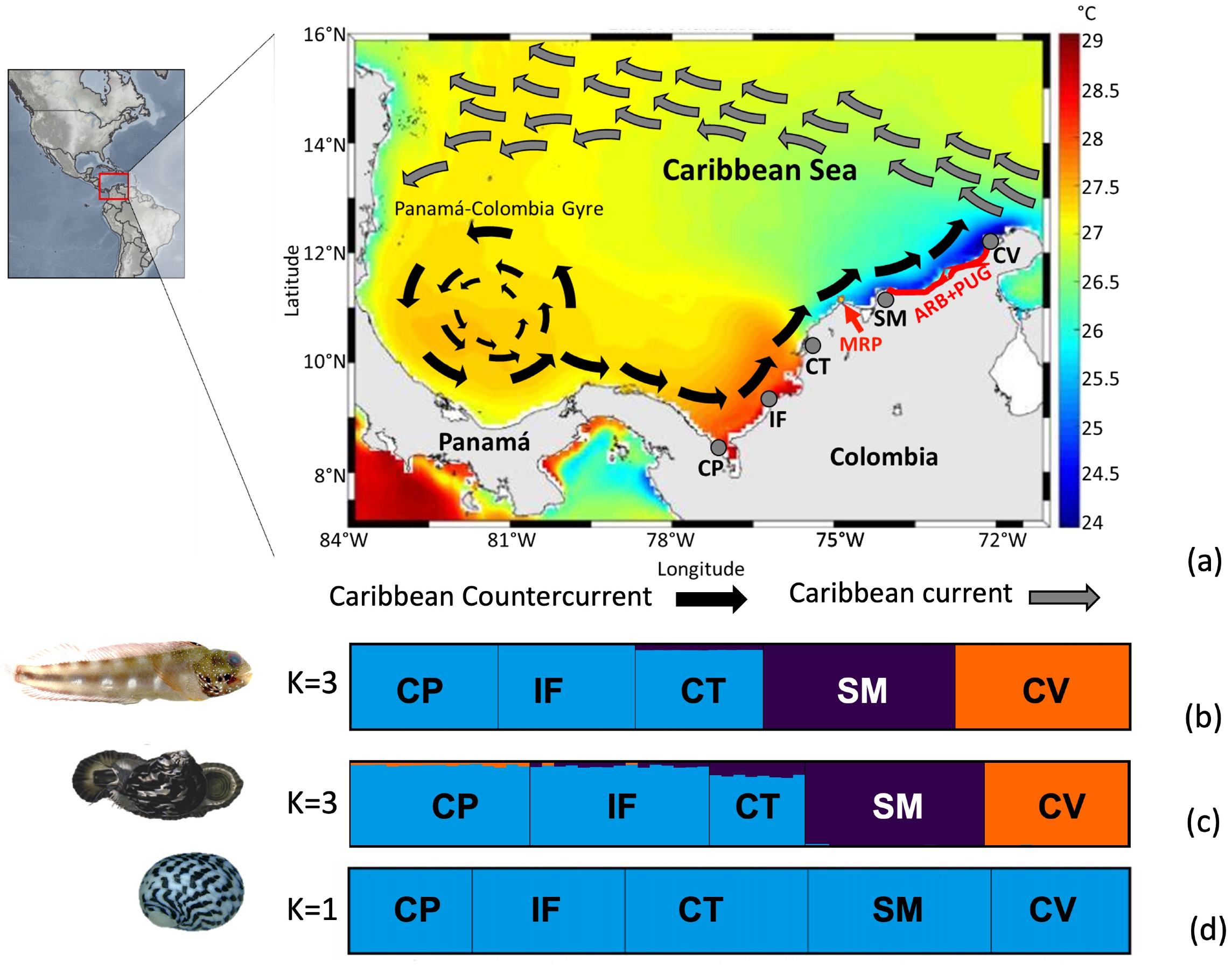The image is a detailed scientific diagram showcasing ocean currents and temperature distribution in the Caribbean Sea. The diagram features a large map, which zooms in on the area around the Caribbean Sea, including Panama and Colombia. The latitude is marked on the left side ranging from 8°N to 16°N, while the longitude is marked on the bottom, ranging from 84°W to 72°W. Temperature in degrees Celsius, ranging from 24 to 29, is indicated on a color scale on the right, with the map itself colored in hues of yellow, green, and blue to depict different temperatures.

The map highlights several currents with black and grey arrows, with black arrows representing the Caribbean countercurrent and grey arrows the Caribbean current. A smaller inset map on the top left shows the Americas with a red square indicating the focused area in the larger map.

Beneath the main map are illustrations of aquatic organisms that resemble slugs and shells, with corresponding blue, purple, and orange tables labeled CP, IF, CT, SM, and CV, indicating K values of 1 and 3. These tables use different colors to possibly categorize data related to the organisms or the currents.

Overall, this detailed diagram provides a comprehensive view of oceanographic conditions in the Caribbean Sea, illustrating currents, temperatures, and possibly marine life distribution.